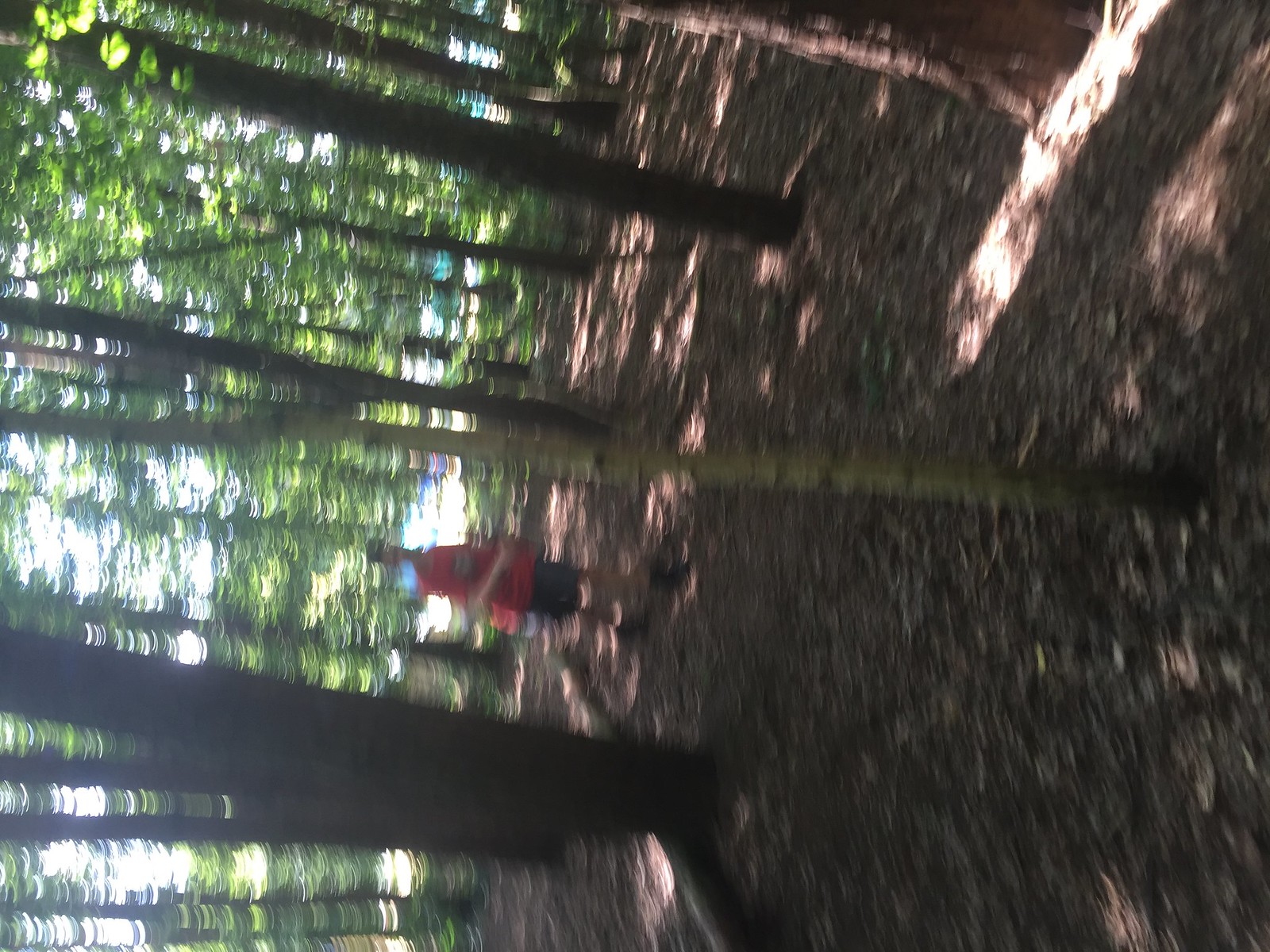The image is a sideways, blurry photograph of a man standing in a forested area. The man, positioned off-center, appears to be in mid-movement, which might explain the overall blurriness of the photo. He is wearing black tennis shoes, black shorts, and a red long t-shirt, possibly adorned with a logo, and may be sporting a black hat and sunglasses, though the blur obscures finer details like facial features. The trees surrounding him are relatively thin, with dark bark, and range from 2-5 inches in diameter. The forest floor is covered in round leaves and appears mulchy. Light filters through the canopy, casting a soft glow and illuminating the deep green foliage above. There is an open field visible behind the man, where the sunlight breaks through more freely, enhancing the natural setting.